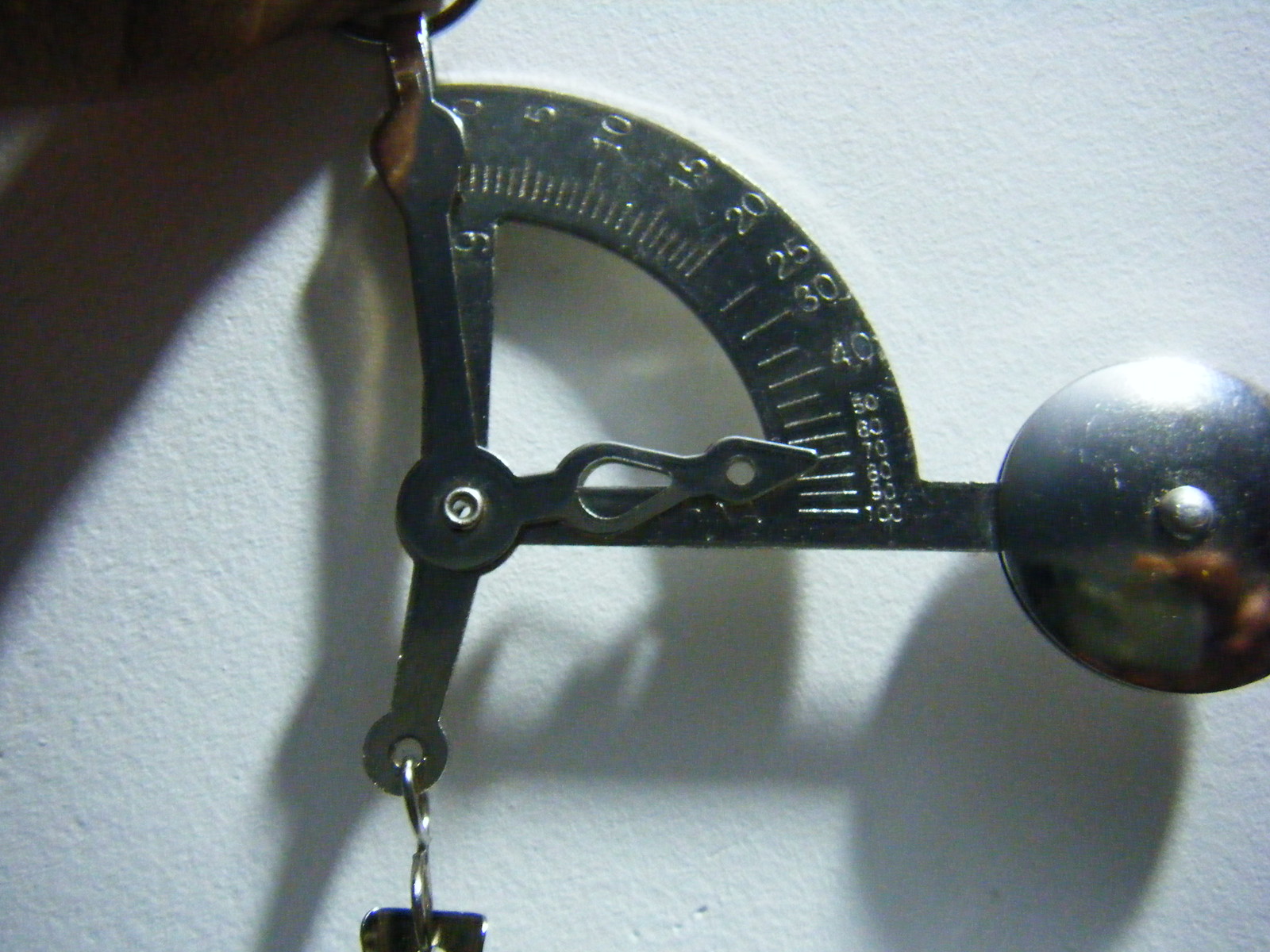The image showcases a detailed metal weighing scale, prominently featuring a measuring tool, likely a protractor. The construction is composed of two main parts: an upright metal rod and an interconnected system of hooks and levers. The rod extends straight up and then bends back down, forming a line leading to a circular pivot point at its center. Attached to this central pivot is another metal rod, further connecting to a weighted mechanism. 

At the bottom, or possibly the side, of this rod is another circle, housing an open ring with a small metal hook. An S-shaped clip is attached to this junction, designed to hold the top of an unseen metal item, likely the weight being measured. 

The protractor, curved in an arch and marked with numerical measurements, is affixed to the upper part of the assembly. The numbers around its edge range from 0 to 100, with larger, evenly spaced numerals between 0 and 40, and smaller increments up to 100. An arrow indicator, centrally located, likely moves in response to the weight placed on the S-clip at the bottom, providing a precise measurement.